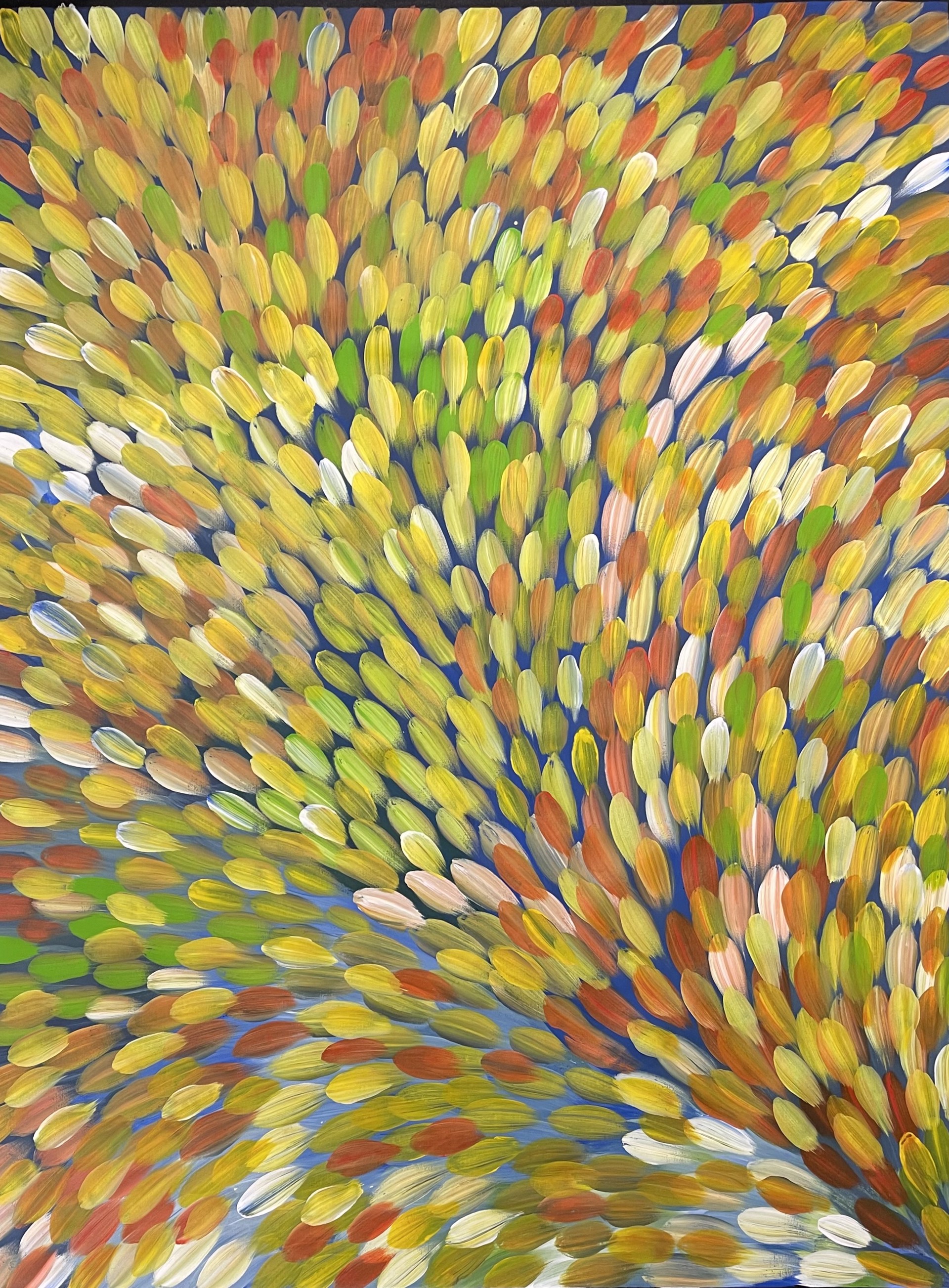The image showcases a vertically oriented painting featuring an array of vivid brush strokes resembling petals or feathers. The primary motif begins in the bottom right corner and radiates outwards, fanning towards the top left, top right, and middle sections. The brush strokes, which are predominantly petal-shaped, exhibit fine stripes indicative of the brush's path. They range in color from vibrant yellows and dark oranges to greens, whites, and subtle peach hues, with yellow being the predominant shade. The background, a contrasting blue, peeks through the multitude of strokes, adding depth to the composition. The strokes' arrangement is dynamic, with some curving up and out to the right, others to the left, and some extending directly upwards, creating a harmonious and lively visual spread.